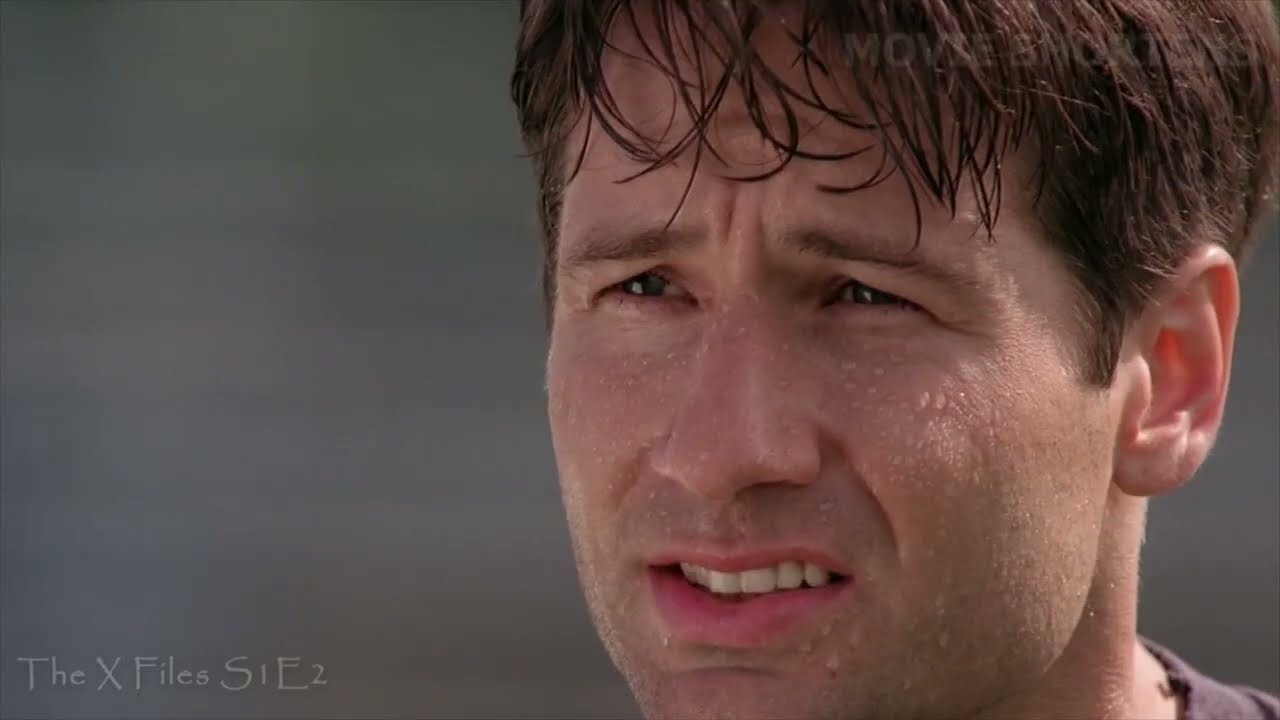The image is a very close-up screenshot of Fox Mulder, a character played by David Duchovny, from the television series The X-Files. Captured from the middle of his forehead down to almost his chin, Mulder's face is off-center to the right side of the image. He has short brown hair slicked with sweat, individual strands visible, and thin brown eyebrows. His frowning expression is accentuated by a furrowed forehead, slightly open mouth showing the top row of his teeth, and his quizzical look. His face is glistening with numerous beads of sweat. The background is blurred and grayish. Mulder is wearing a brown t-shirt, with only a small part of his shoulder showing at the bottom right. The lower left corner of the image contains the text: "The X-Files, Season 1, Episode 2."